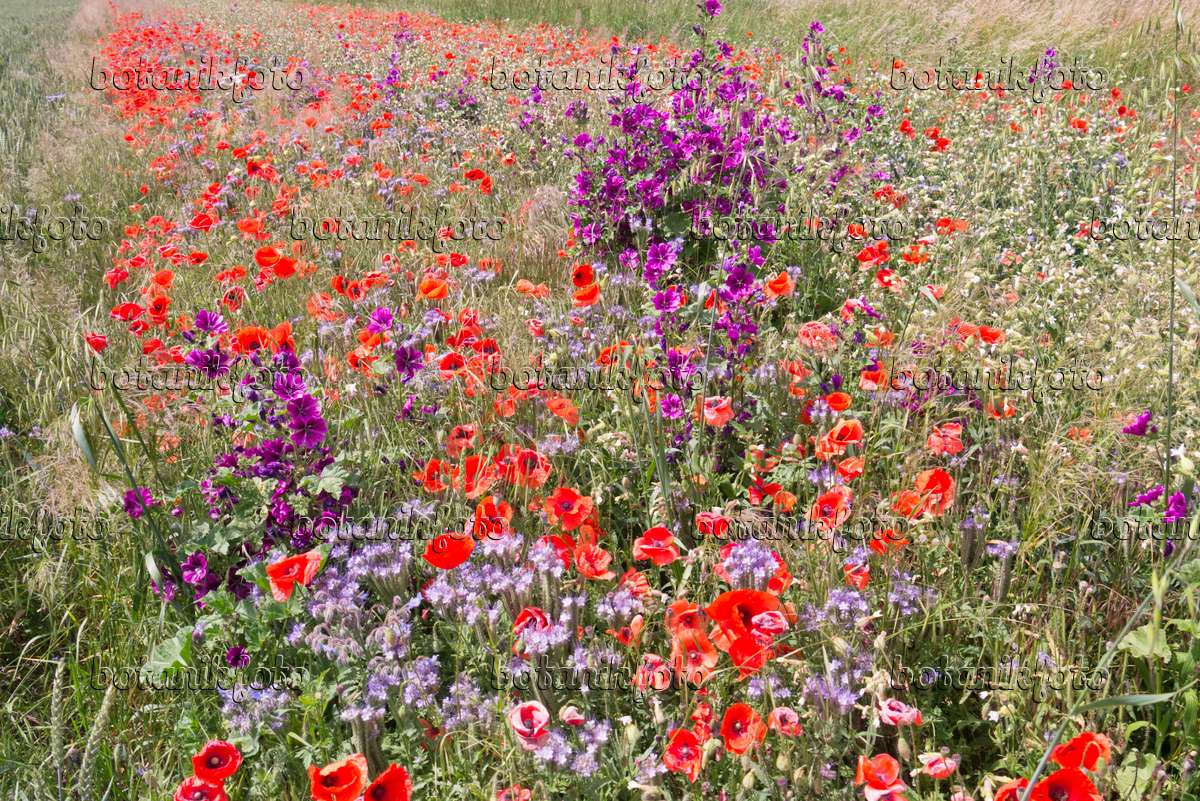A vibrant photograph captures a wild field of dense, multi-petaled wildflowers in full bloom, with an almost endless expanse of striking colors ranging from tangerine and salmon to lilac, pink, violet, and interspersed whites and grays. In this sea of color, a few yellow blossoms and surrounding seed-bearing grasses blend seamlessly. The tallest flowers gather at the center, forming a bouquet-like arrangement of violet blooms. Various types of weeds and grasses are intermingled, adding to the natural, untamed beauty of the landscape. Despite the vivid detail of the flowers, which include red poppies and possible asters among the mix, the image is overlaid with multiple embossed watermarks in several rows from left to right, making the lettering difficult to read but indicating the photo originates from a stockhouse, likely named Botanic Photo. The movement of the wind can almost be felt through the subtle blur of the greenish-gray grasses on the peripheries of this captivating scene.